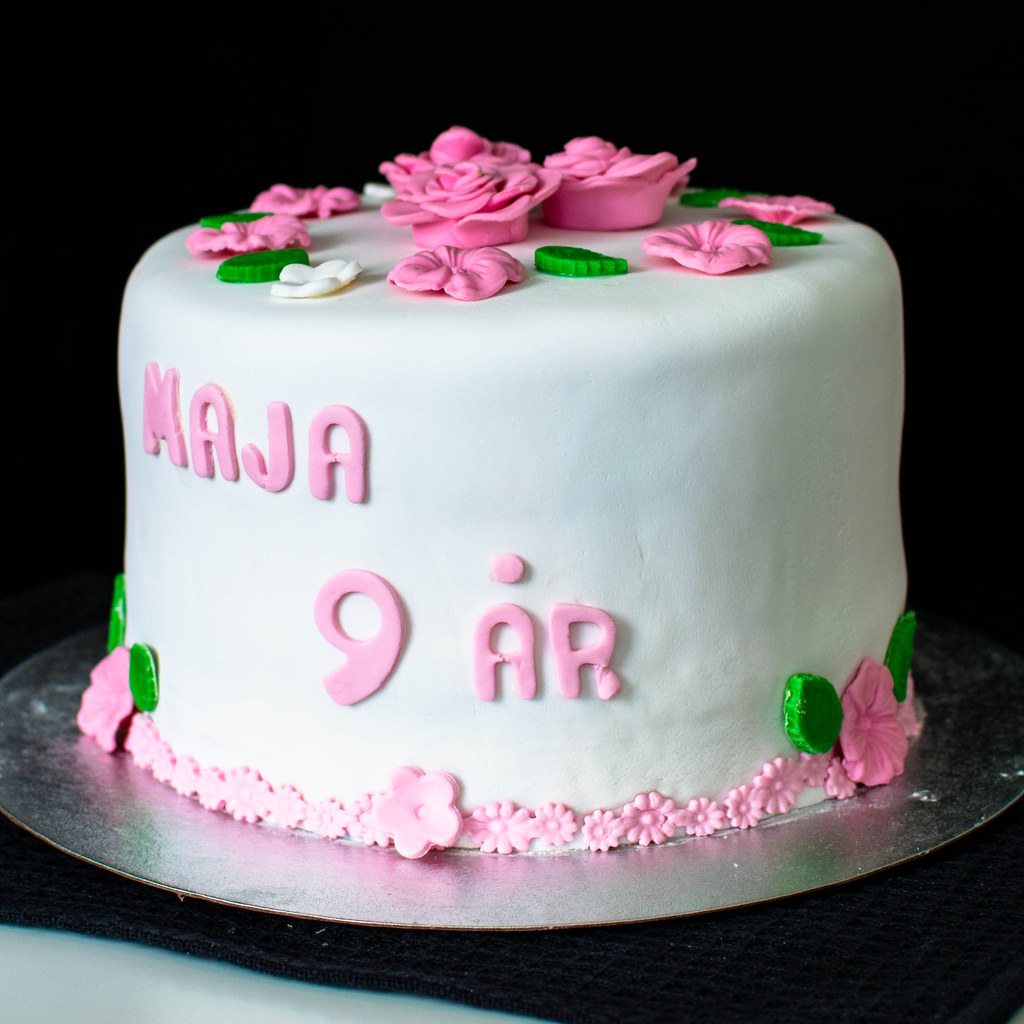The image is a close-up, color photo of a meticulously decorated cake under bright light with a pure black background. The cake is displayed on a round, reflective silver disc, likely a cardboard cake board coated with what looks like aluminum foil. A small portion of a white table or surface, possibly covered by a dark tablecloth or placemat, is visible in the lower left corner.

The cake itself is tall, likely consisting of two or three layers, and is uniformly coated with a solid, white fondant. Intricately crafted pink and green decorations adorn the cake, with the side displaying the text "MAJA 9ÅR" in well-defined pink frosting, indicating a celebration for Maja's ninth birthday. 

The top of the cake boasts an elaborate arrangement of pink rose decorations made of the same type of frosting, complemented by small white flowers and green, serrated leaves. Around the base, the cake features a chain of pale pink daisy-shaped flowers of varying sizes, with medium-sized flowers flanked by large flowers positioned on the left and right. Each large flower is adorned with green leaves, adding to the lush, floral theme of the decorative confection.